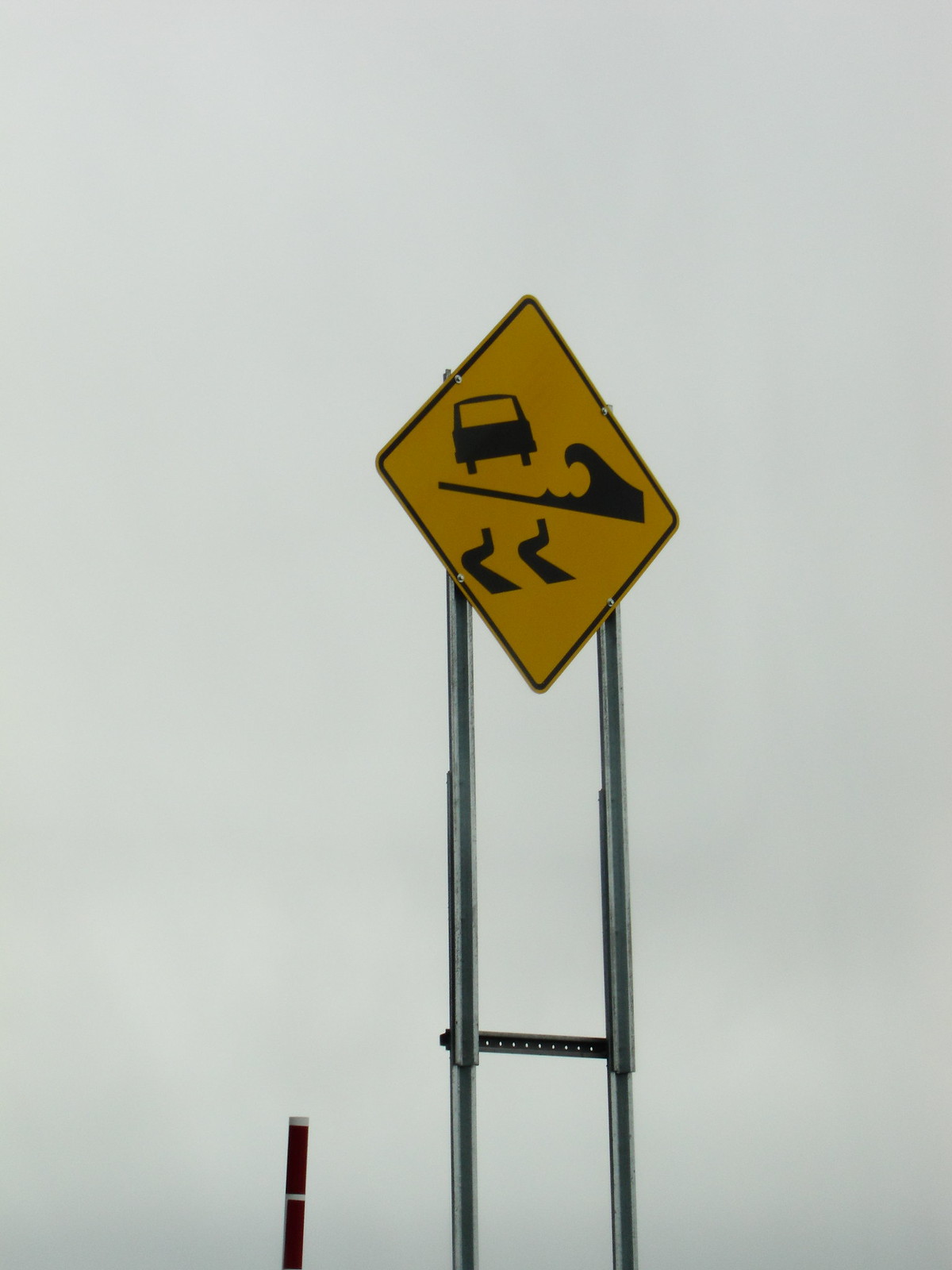A computer-generated image depicts a detailed street sign against a light gray background. Starting from the bottom left corner, there's a small pole featuring a brown shaft with a white tip. The central portion of the image showcases two overlapping grayish bars, bolted together, and stabilized by a crossbar pierced with evenly spaced holes. At the top of this structure is a rectangular yellow sign, oriented diagonally so that its tips form a diamond-like shape. The sign displays a black silhouette of a car viewed from the rear, with a curvy line beneath it representing a road, accompanied by a wave of water and wavy tire marks below the line. This imagery suggests the message "Slippery When Wet."